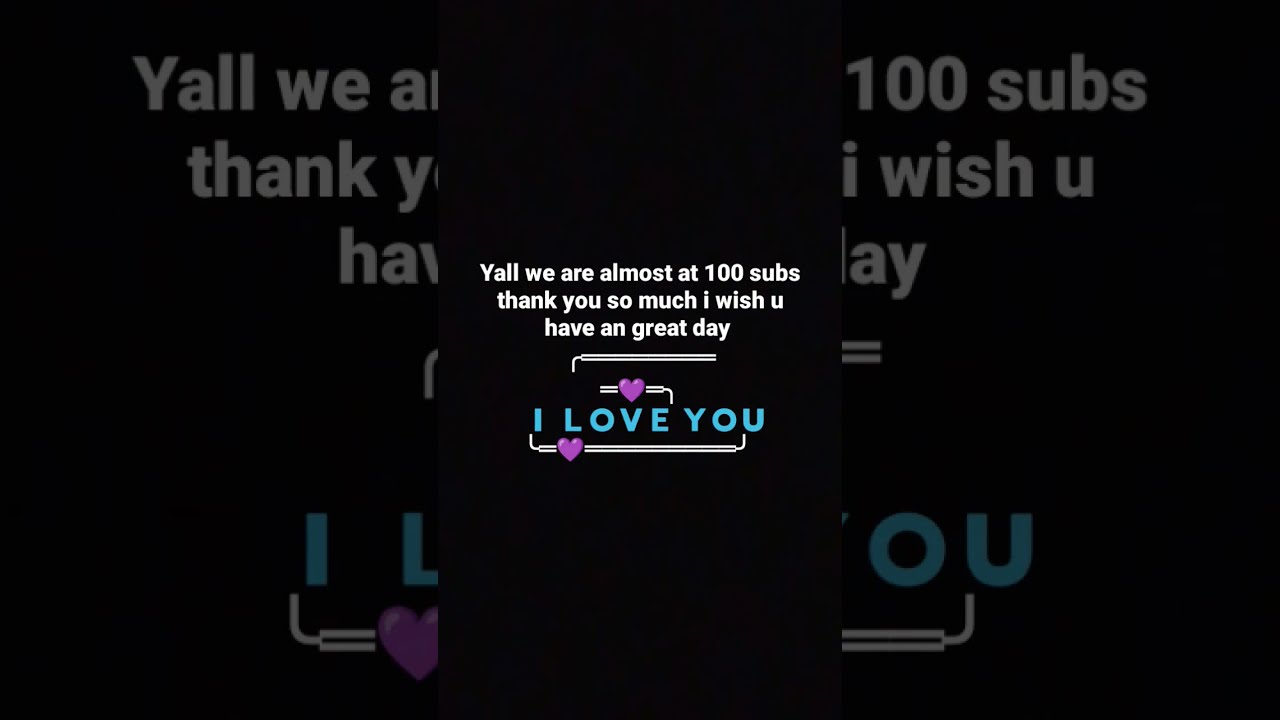The image features a predominantly black background with three sections. The central section stands out with bright white text, reading: "Y'all, we are almost at 100 subs. Thank you so much. I wish you have a great day." This text is separated by lines interlaced with purple hearts. Below, in bold blue letters, it says "I LOVE YOU," also accented with pink hearts. The left and right sections of the image are faded renditions of the central portion, serving as a border. The overall composition of the image resembles a high-definition television screen, focusing attention on the central message.